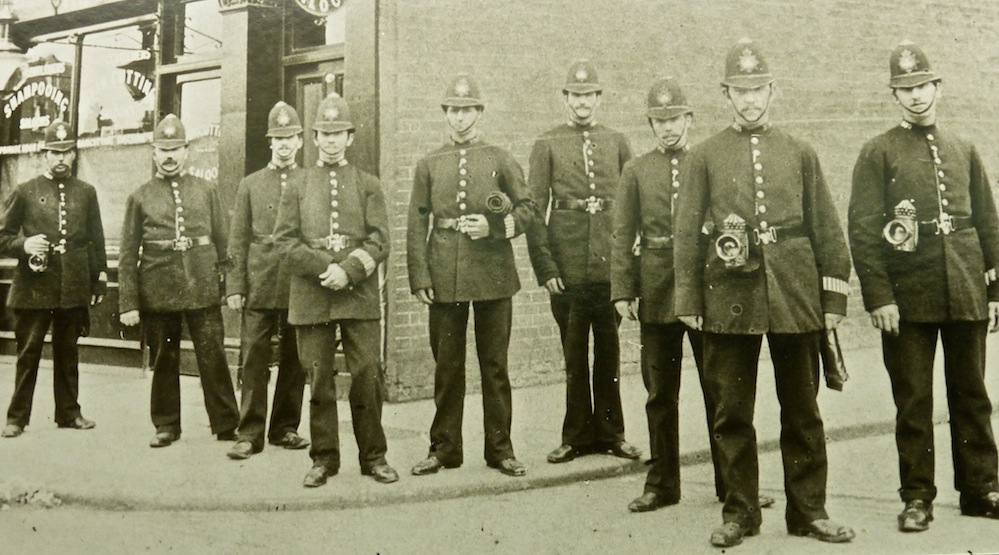This is an old, grainy black-and-white vintage photo depicting a group of about nine men in uniform, standing on a sidewalk in front of a brick building, possibly a storefront or a restaurant. The men appear to be servicemen, potentially policemen or firemen, based on their attire and the equipment they are carrying. They are wearing identical dark uniforms consisting of a long coat with light buttons, dark pants, and belts around their waists, which seem to have metal canisters attached, possibly flasks or other equipment, marked with a circular emblem on the front. Each man has a hat with a prominent starburst badge and a strap under the chin. The group is not perfectly aligned and poses in a slightly disorganized manner, yet they all look straight ahead, giving a sense of the historical and formal nature of the moment captured.